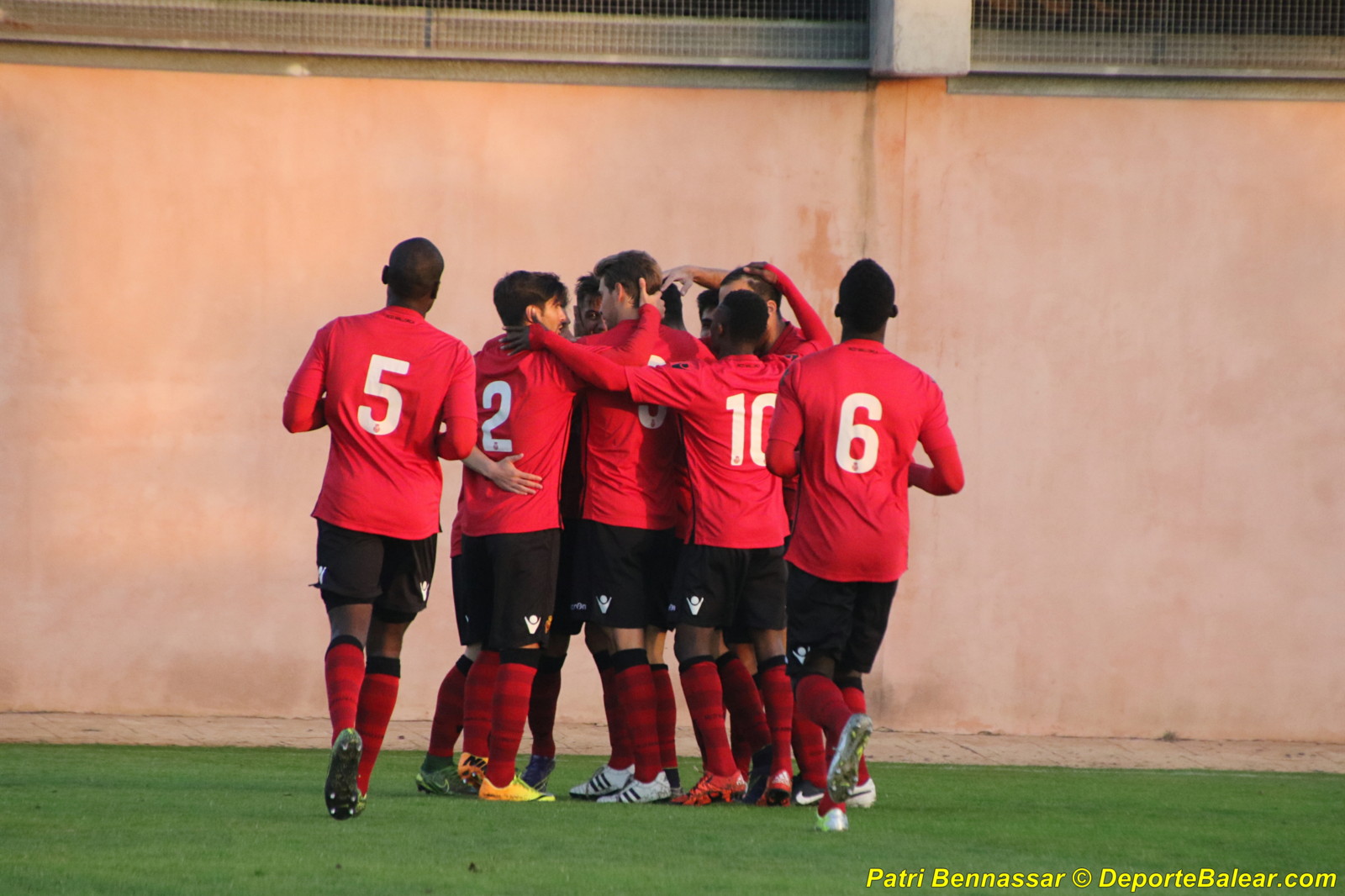In this vibrant daytime photograph, a team of soccer players is huddled together at the center of a flat, grassy field. They are all embracing and patting each other on the head, creating a display of camaraderie. The players are all facing away from the camera, making visible the numbers on their red jerseys—specifically, numbers 2, 5, 6, and 10. They are dressed uniformly in long-sleeve red shirts, black shorts, red socks with black tops, and soccer shoes. Surrounding the green field is a light pale coral-colored concrete wall, topped with metal netting. The top portion of the image captures additional details of the sidewalk and another stone wall. In the lower right-hand corner, the text "Patry Benasar, copyright DeportBellier.com" is visible in yellow, marking the creator's credit. The overall scene captures a moment of unity and support among the players in a well-defined outdoor soccer field setting.